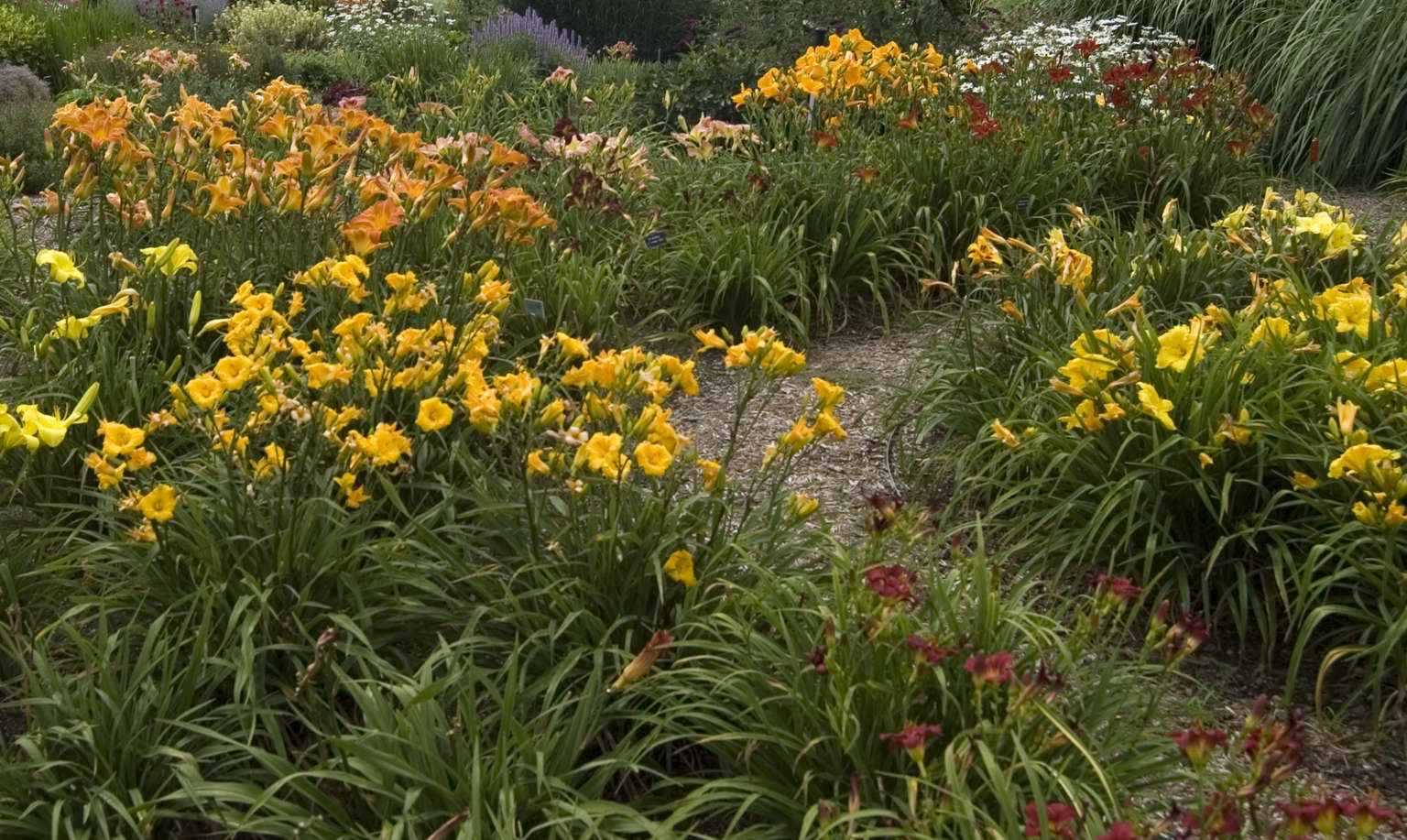The photograph depicts a vibrant, lush field of wildflowers in a well-maintained green space, likely during spring or summer when everything is in full bloom. In the bottom right corner, there's a bush of tall, long-leaved red flowers. A gravel pathway extends in a V-shape from the lower right corner toward the upper right, creating a natural division among the flowers. On the picture's right-hand side, yellow bell-shaped flowers can be seen, rising gracefully amidst the greenery. Toward the middle and left side of the image, clusters of orange, pink, red, and white flowers are scattered, each on high stalks. In the background, the greenery stretches further, dotted with more colorful blooms. The scene exudes a tranquil and picturesque atmosphere, capturing the essence of a thriving garden space.